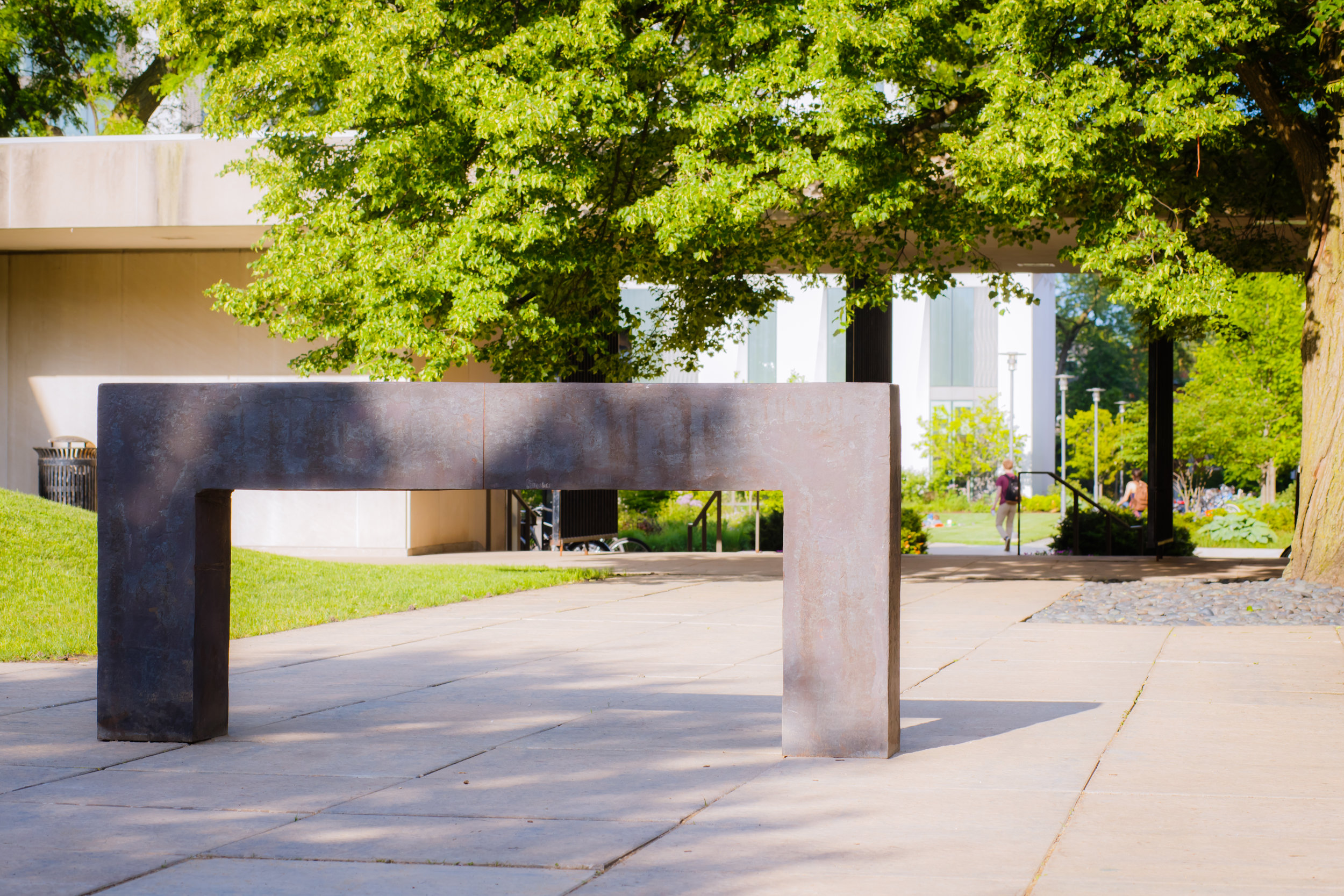The image depicts a modern outdoor sculpture that stands prominently in the center of a vertical rectangular frame. This sculpture consists of two vertical, parallel concrete slabs that are connected at the top by a horizontal slab, forming a square archway approximately five feet tall. The sculpture is a minimalist piece made of gray concrete and is set on a broad, flat concrete walkway. The background reveals a park-like setting with green trees, a concrete wall about 10 feet high with an overhanging roof, and a concrete path that opens at the center, allowing passage. Beyond the sculpture, the park extends with visible elements including a bridge or overpass partially obscured by trees, some stairs leading to a lower section of the park, and a tall white building in the far distance. There are a few people walking along the pathways in the background. On the left edge of the image, a small grassy hill and a trash can are visible, adding more detail to the setting. The photo is taken in bright, natural light which enhances the clarity and details of the scene.